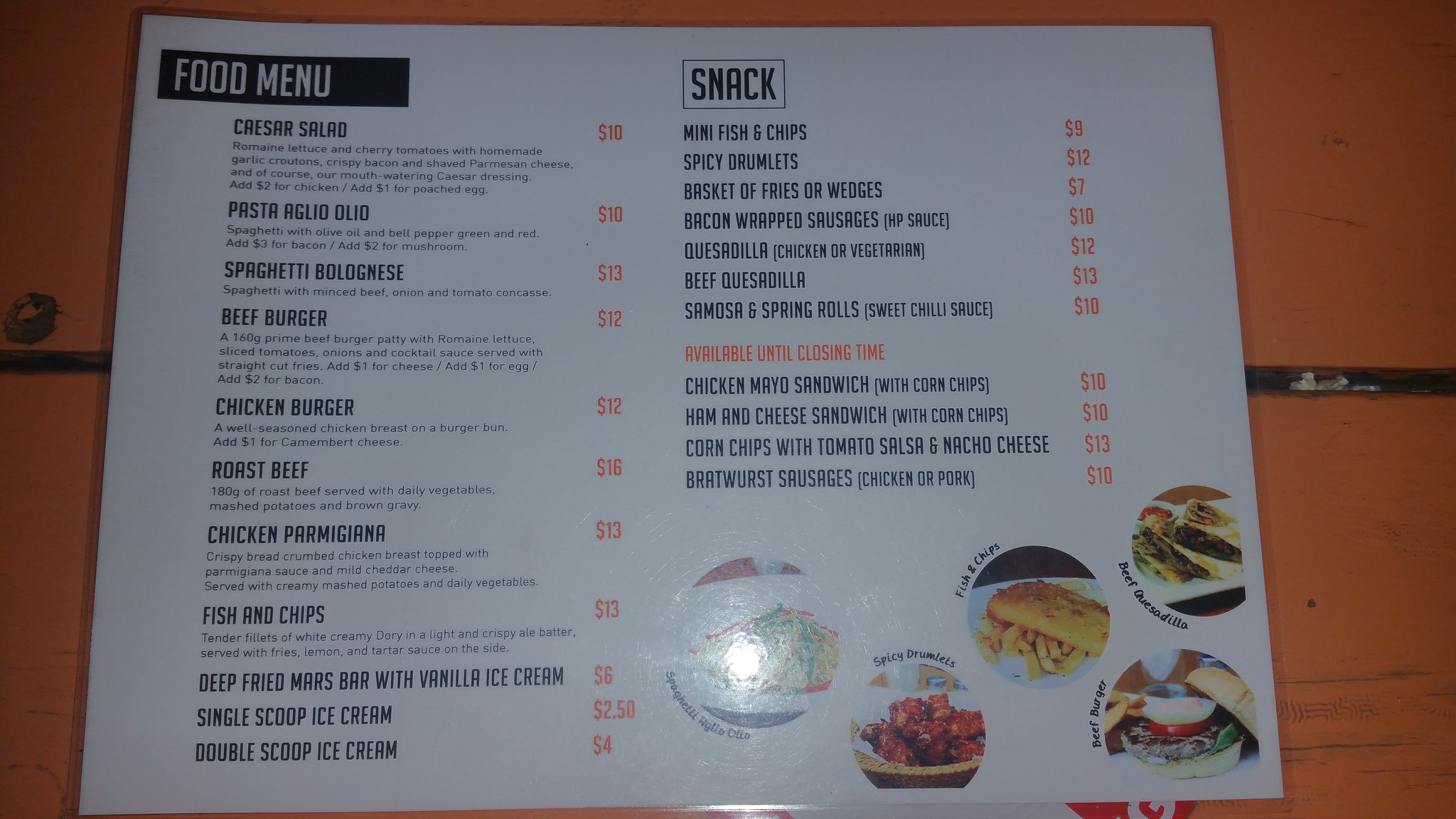A large laminated food menu is displayed on an orange surface with a black seam running through it. The menu is titled "Food Menu" and features a variety of dishes, organized into categories.

**Entrees:**
- Caesar Salad
- Pasta (Spaghetti Bolognese)
- Beef Burger
- Chicken Burger
- Roast Beef
- Chicken Parmesan
- Fish and Chips
- Deep-Fried Mars Bar with Vanilla Ice Cream

**Desserts:**
- Single Scoop of Ice Cream
- Double Scoop of Ice Cream

**Snacks:**
- Mini Fish and Chips
- Spicy Rumlets
- Basket of Fries or Wedges
- Bacon-Wrapped Sausages
- Quesadilla (Beef Quesadilla)
- Samosa
- Spring Rolls

**Sandwiches:**
- Chicken Miro Sandwich
- Ham and Cheese Sandwich
- Corn Chips with Tomato
- Brockwurst Sausages

The menu lists the items in black text, with prices highlighted in red. At the bottom, there are images showcasing some of the dishes. The offerings are available until closing time.